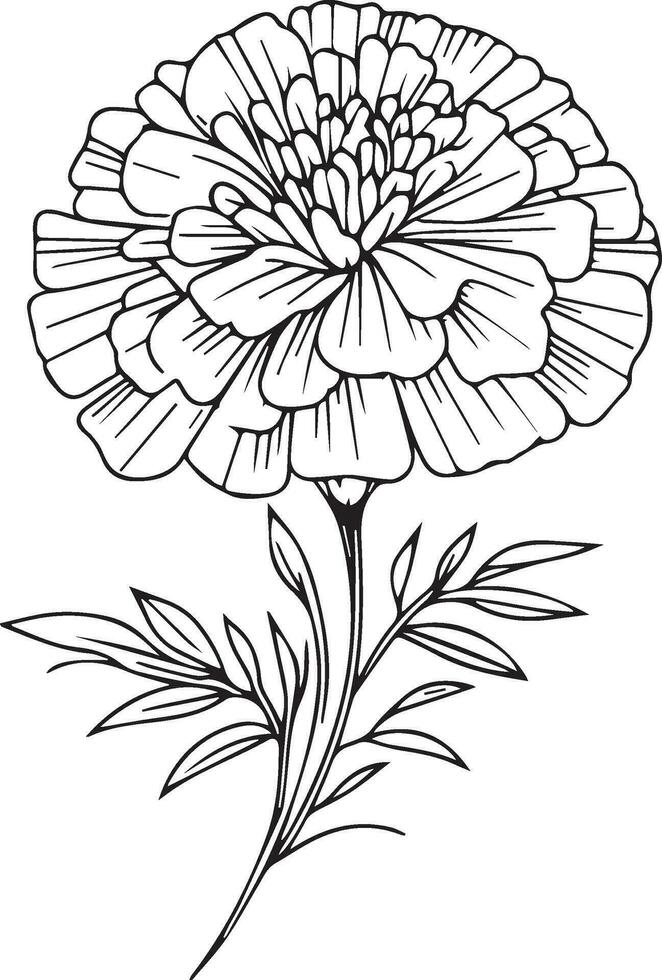The black and white line drawing features a detailed flower, likely a carnation or chrysanthemum, positioned prominently in the center of the image. Rendered in a simple, modern pen and ink style, the drawing showcases the intricacies of the petals, each petal distinctly delineated to convey texture and structure, with numerous lines hinting at the natural creases and folds. The flower's stem is thin and extends outward, accompanied by several branches of leaves with their own detailed lining. While flat and without shading or depth, the image conveys a basic yet beautiful design suitable for coloring, resembling templates often found in coloring books. Overall, it’s a close-up view emphasizing the plentiful petals and the delicate, simplistic elegance of the flower.